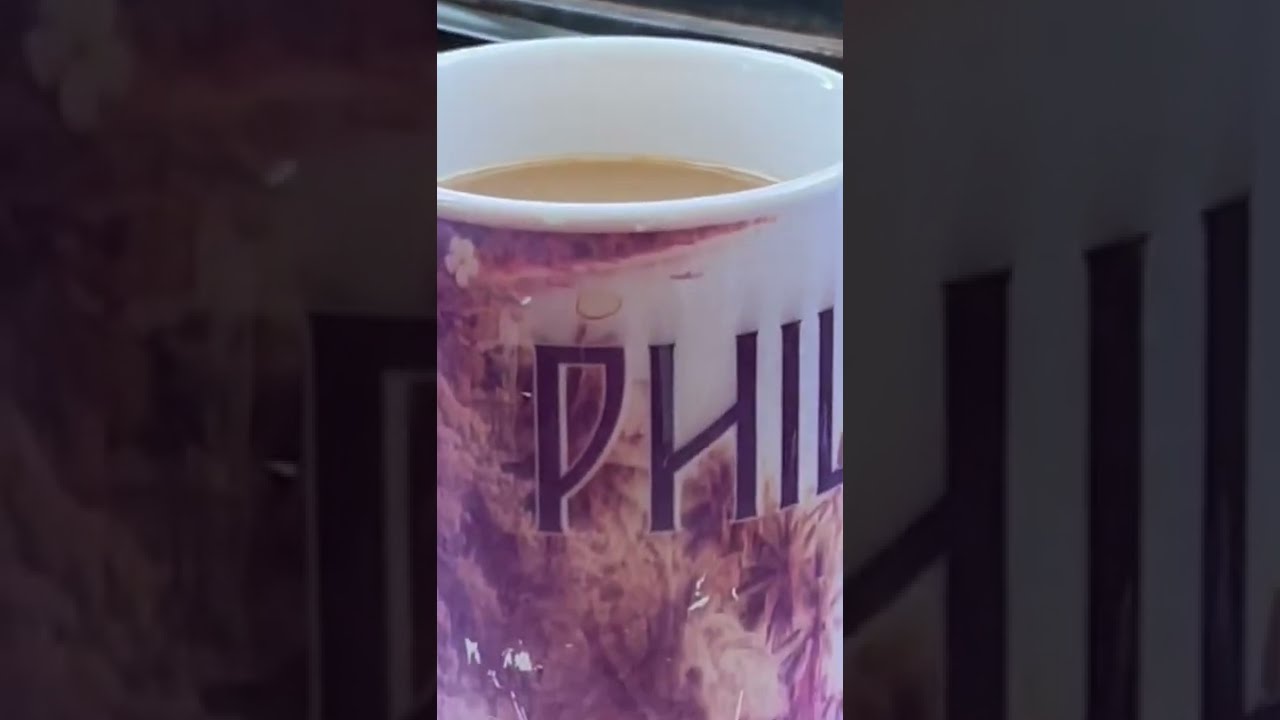The image is a detailed and segmented photograph of a coffee mug filled with light brown coffee, likely with some cream. The mug is white with a nature-inspired design that includes green and beach-like elements, and prominently features the word "PHIL" in bold, black capital letters across its surface. The overall layout of the photograph is a horizontal rectangle with a central vertical rectangle clearly showcasing the coffee mug. The segments flanking the central image are darkened and blurry, appearing as if a filter has been applied. These side segments are zoomed-in portions of the coffee mug itself, emphasizing the design and the text even in their obscured state. The combination of these elements creates a unique and artistic composition, highlighting the central coffee mug amidst a creatively blurred, filtered background.